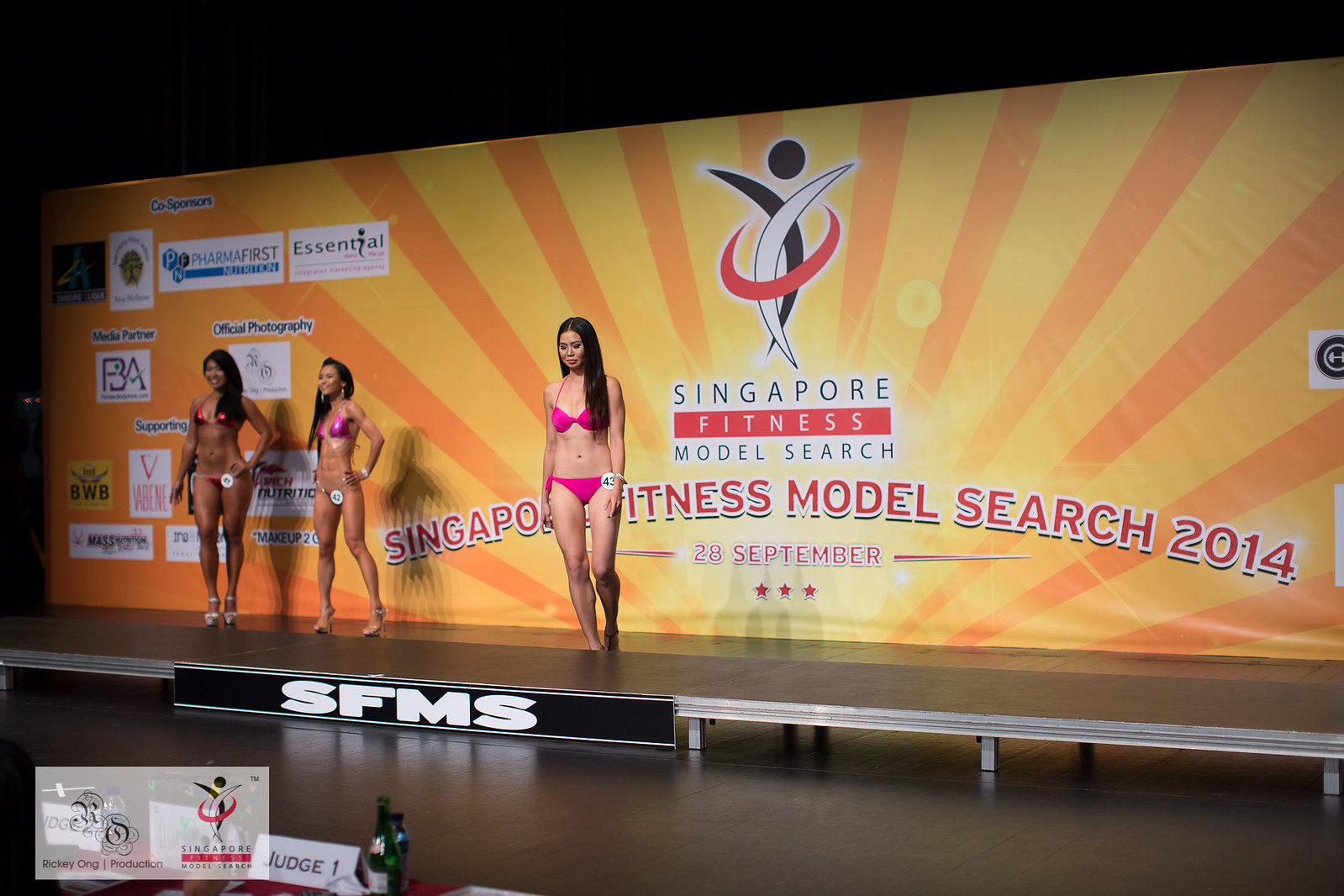This photograph captures a vibrant scene from the Singapore Fitness Model Search 2014, held on 28 September. Center stage are three Asian women walking confidently in bikinis, showcasing their physiques in front of a keen audience. The woman in the middle wears a striking pink bikini, while the two women flanking her are dressed in red bikinis, each with long black hair styled elegantly. 

Behind them, a large backdrop dominates the scene with an intricate black, white, and red design featuring a round black circle at the top. This design cradles the event's name, "Singapore Fitness Model Search," boldly displayed twice. Below it, the date "28 September" and three red stars are prominently shown. The background also includes a semi-circular arch emblazoned with "Singapore Fitness Model Search 2014."

To the right are various sponsor logos, including one marked "BA" and another for "Essential." At the lower left, the letters "SFMS" (Singapore Fitness Model Search) stand out on the stage, along with placards indicating the judge's positions, one labeled "Judge 1." Notably, a bottle of wine can be seen on the judge’s table, adding a distinct touch to the glamorous setting.